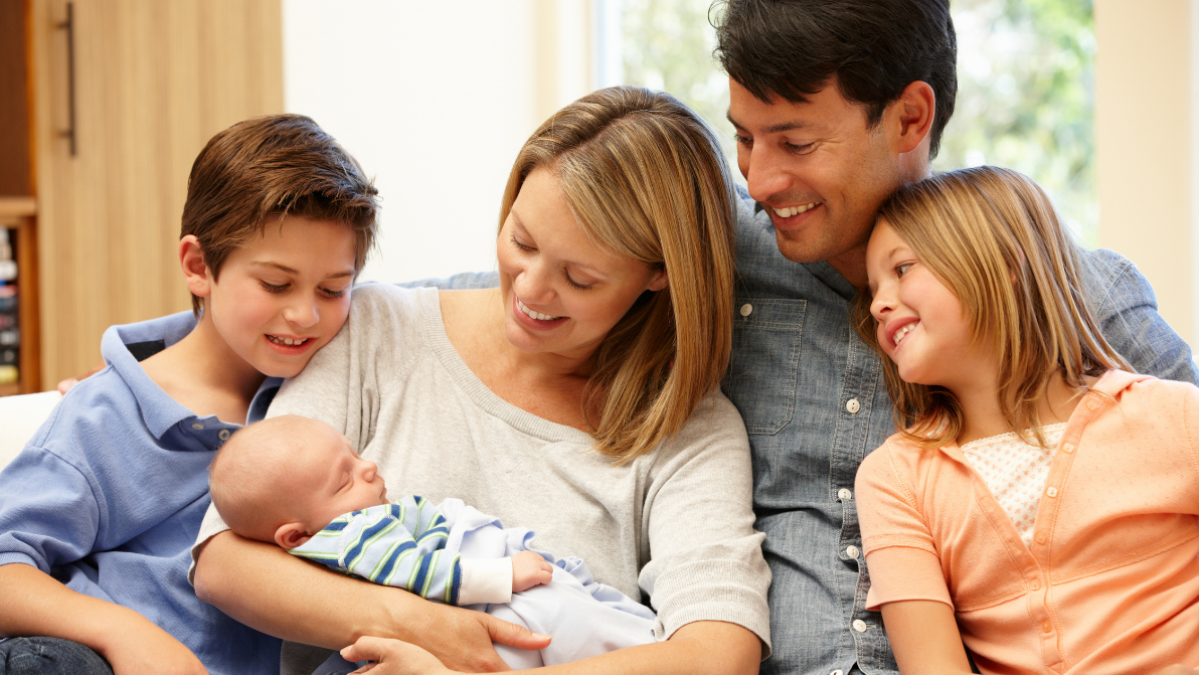This detailed family portrait, potentially taken for an advertisement, captures a loving family of five in a studio setting with bright, out-of-focus background lighting. At the center, a mother in a light grey sweater lovingly holds a newborn dressed in a green and grey striped shirt and covered with a blue blanket. She gazes down at the baby with a warm smile. To her right, a young boy, around eight years old, leans on her shoulder, also smiling at the baby. Beside him is the father, wearing a blue denim shirt, embracing the entire family and looking adoringly at the newborn. On the right side of the image, their older daughter, likely between ten and eleven years old, wearing a peach-colored shirt layered with a white one dotted with patterns, leans against her father and also focuses intently on the baby. In the background, partially visible furniture, a handle that opens a door, a stack of books or movies, and some green leaves add depth to the composition. All family members exhibit expressions of admiration and joy, forming a heartwarming and cohesive family unit centered around the newest addition.